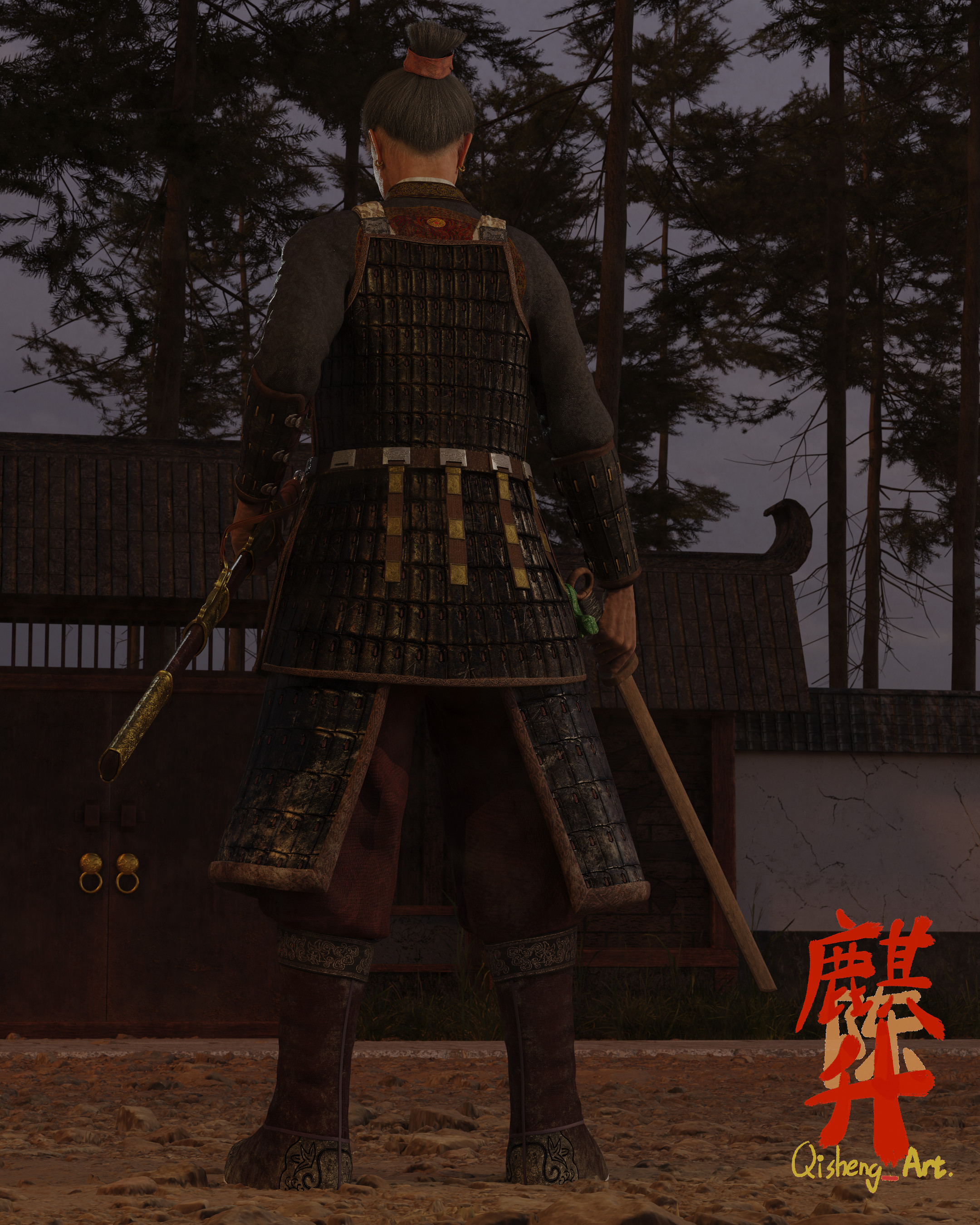The image depicts a person who resembles a samurai, with their back facing the viewer. They stand in the midst of a traditional Eastern Asian courtyard, with large trees visible in the background. The individual has light skin and brown hair styled in a bun. They are dressed in a long-sleeve gray shirt with protective cuffs extending from elbow to wrist, a black garment that appears to be a dress or tunic, brown pants, and brown boots. They hold a wooden weapon in one hand and its sheath in the other. The scene appears to be set on a dirt ground, possibly within an outdoor arena. At the lower left corner of the image, there are some Asian characters, followed by the phrase "Key Shing Art" or similar. The image has a dark, slightly mysterious ambiance, potentially suggesting it was created digitally for a video game.